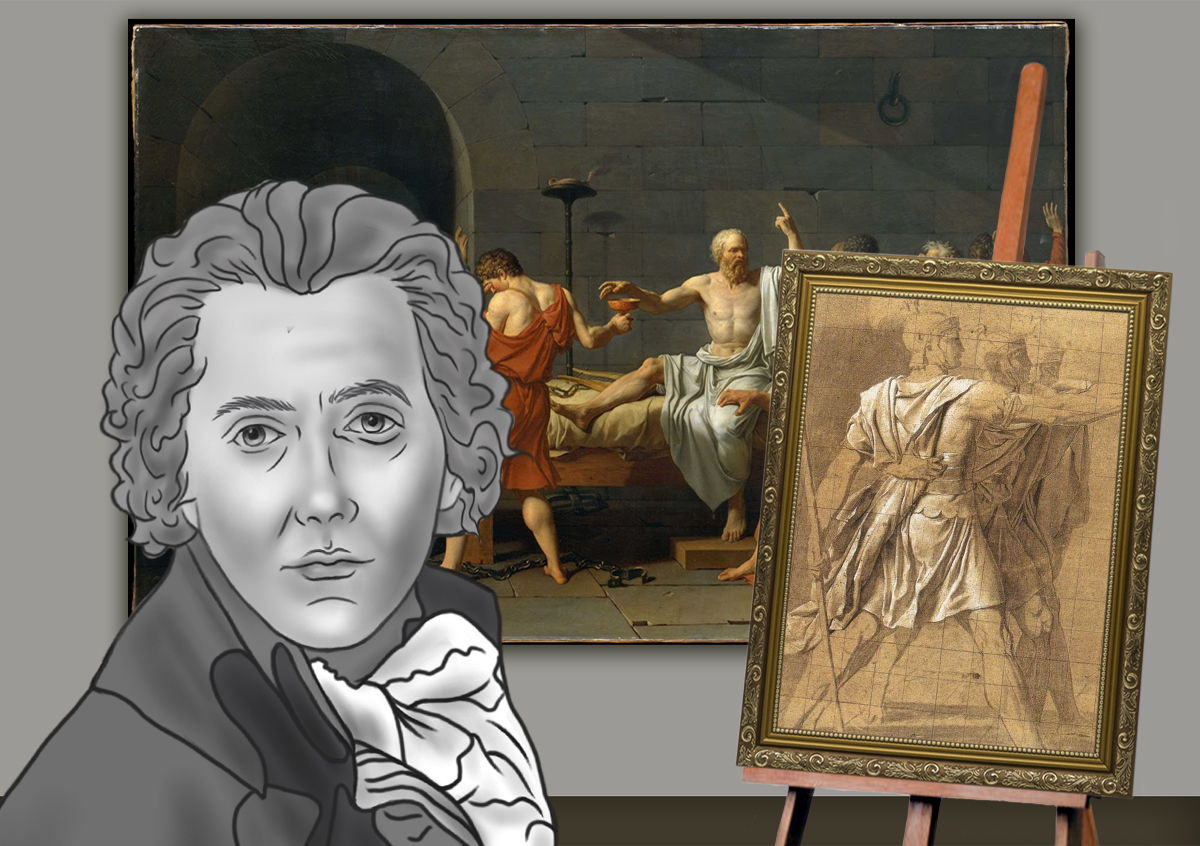In the image, a detailed scene unfolds with several layers of artwork. In the front lower left corner, there is an intricate illustration of a man dressed in 1700s colonial attire. He has swept-back hair, just below his ears, and is wearing a dark jacket with a poofy white necktie. His light eyes and clean-shaven face gaze directly at the viewer, commanding attention. Behind him, an ornate gold-framed artwork rests on an easel, showcasing a meticulously detailed brown and white pencil drawing. This drawing depicts two Roman soldiers in armor, their faces masked, with one extending an arm holding a long, narrow weapon, standing in front of a rugged rock wall. In the background, a large painting dominates the wall, showing a dramatic scene where a man in a luxurious orange robe is tending to a person in a white robe, both surrounded by attendants—hinting at a royal figure possibly in distress. The juxtaposition of these diverse artworks creates a rich, multi-layered visual narrative, blending various historical and artistic themes.